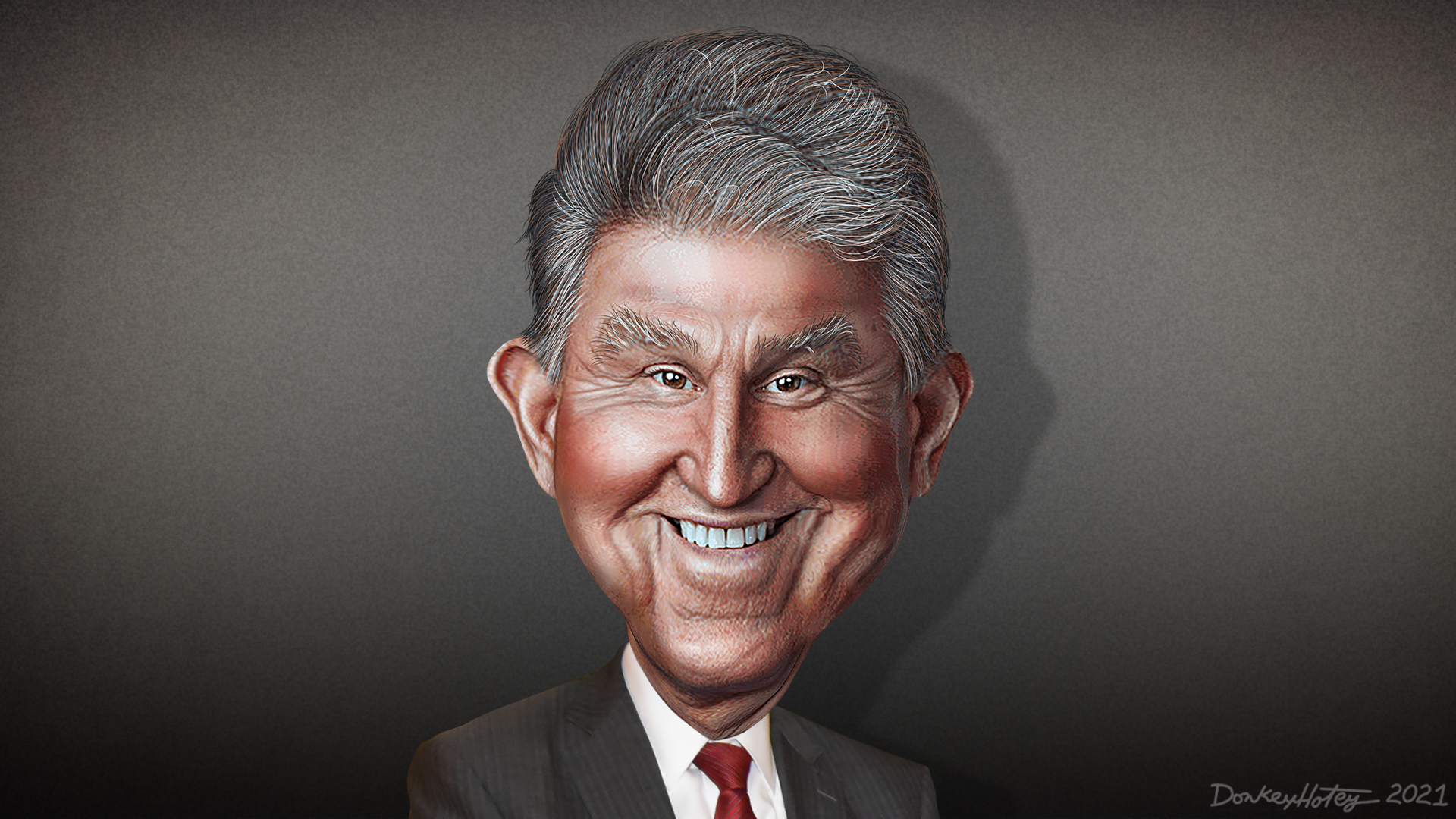The image features a detailed caricature of an older man with salt-and-pepper gray hair and bushy eyebrows, captured against a light gray background that gradually darkens towards the corners. His head is exaggeratedly large, with small brown eyes, large ears, and realistically rendered teeth visible in a broad, cheerful smile. The man has a light tan complexion and is depicted wearing a gray pinstripe blazer over a white button-down shirt, accessorized with a dark red tie. A subtle head shadow falls to his right. In the bottom right corner, the signature "Donkey Hotey 2021," written in light gray cursive, is visible, identifying the artist or the work's title.